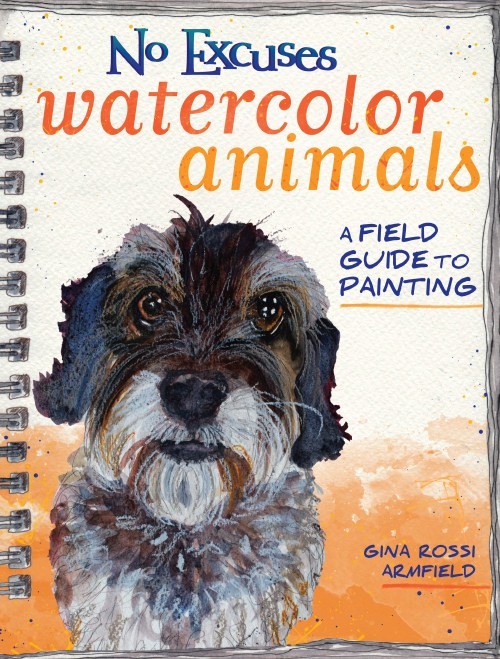The image showcases the cover of a spiral-ring-bound book titled "No Excuses, Watercolor Animals: A Field Guide to Painting" by Gina Rossi Armfield. The cover features a watercolor painting of a small European dog, possibly a Schnauzer, with an expressive gaze. The dog is depicted in shades of black, gray, brown, and white, with the background painted in warm hues of orange, darker orange, and white. The title features various colors: "No Excuses" in blue, "Watercolor Animals" in two shades of orange, and "A Field Guide to Painting" in dark blue with a yellow-orange underline. The overall design suggests a well-loved, vintage appearance, hinting at the book's enduring use.